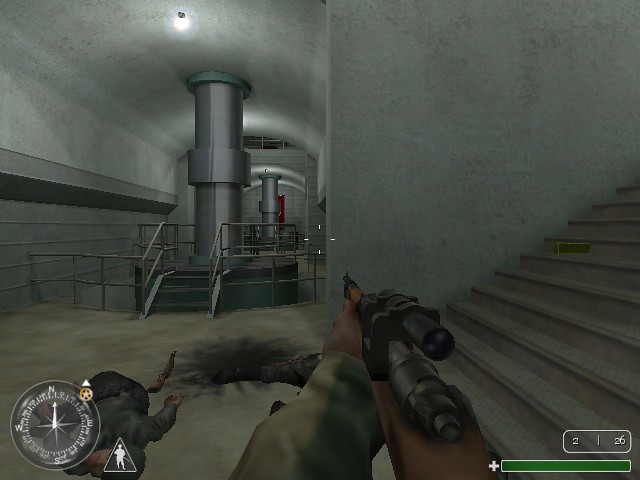This black-and-white image appears to be a screenshot from a first-person shooter video game, capturing a moment within a cave-like environment. In the bottom left corner, a compass displays the needle pointing north. Adjacent to the compass, there is an icon depicting a white silhouette of a soldier. The top right corner of the screen features a rectangular box showing the figures "2/26". Below this, another long rectangular box, filled predominantly with green and marked by a white cross on its left side, is likely indicating the player's health status. Dominating the foreground, the perspective showcases the player's hands gripping a machine gun, complete with a visible scope mounted on top of the rifle. The immersive first-person view suggests the character is navigating through a cave or tunnel within the game.